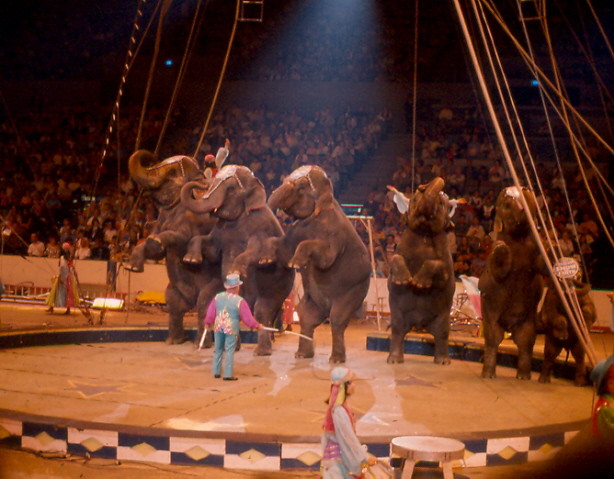In the bustling atmosphere of a colorful Three Ring Circus, a captivating scene unfolds in the center ring where six elephants, five adults and one baby, stand proudly on their hind legs in a disciplined formation. Each elephant is adorned with a decorative headdress, adding to the grandeur of the spectacle. The tallest elephant stands on the left, progressively getting smaller toward the right. Commanding their attention is a ringleader, dressed in a striking ensemble comprising blue jeans-like pants, a pink long-sleeved shirt, and a bluish embellished vest, topped with a blue top hat. He holds a white wand or stick in each hand, directing the impressive act with precision. In the foreground, a figure dressed in a flowing, Arabic-inspired outfit in shades of blue, pink, and yellow, reminiscent of Princess Jasmine, walks across the ring carrying a tambourine. Above the scene, strings and wires descend from the ceiling, framing the performance without obscuring the view. Behind the elephants, an eager audience fills the stadium seating, captivated by the magnificent display.